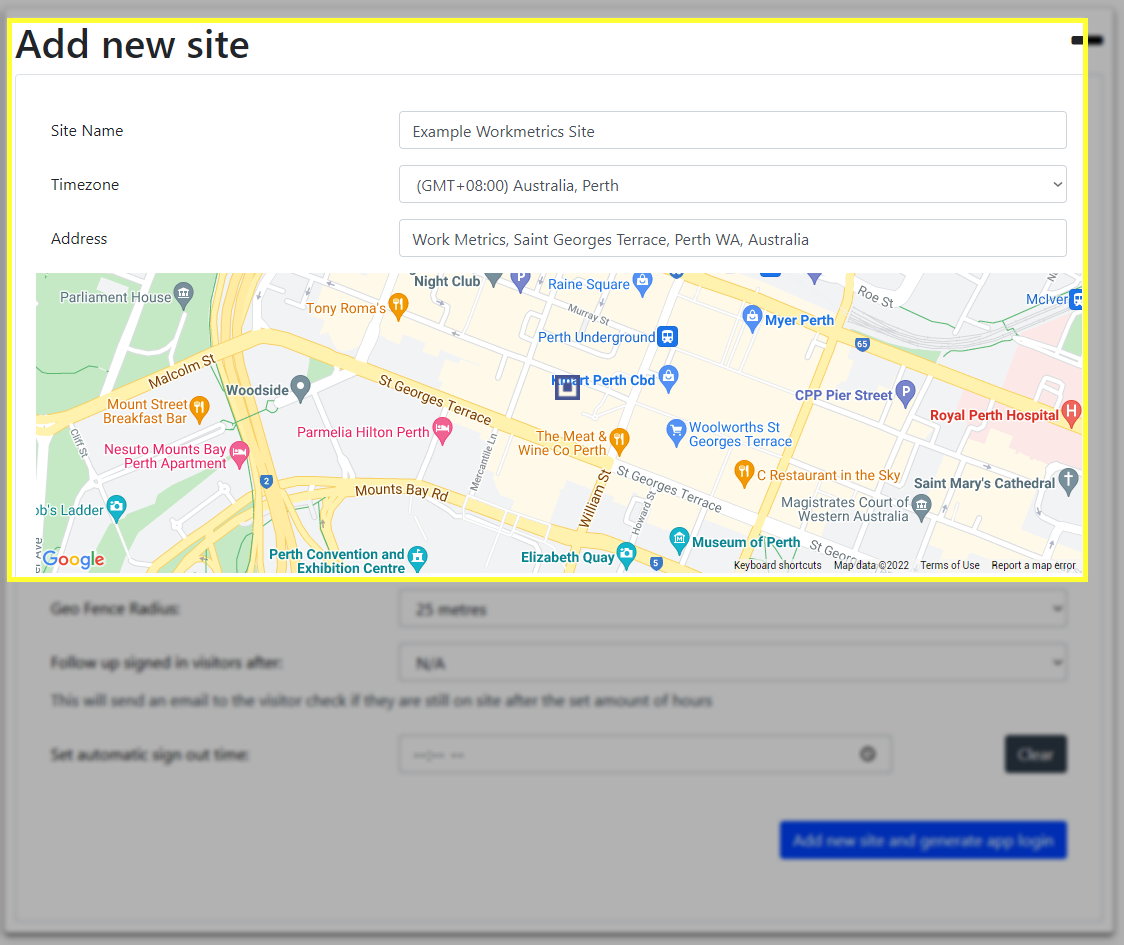The image appears to display a screenshot of a Google Maps interface centered on Perth, Western Australia. The map highlights various landmarks including St. George's Tower, Parliament House, Mount Street Breakfast Bar, The Suite on Mount, Spade Perth Apartments, Parmelia Hilton, Tony Roma's, Green Square, Perth Underground, Meet and Wine, and Sea Restaurant and Sky at St. Mary’s Cathedral. Also noted are the Hospital Museum of Perth, Elizabeth Quay, Perth Convention and Exhibition Center, and the central business district (CBD). The background of the image is blurred, showing a form with fields that seems related to creating a website or adding a new site. There are options visible to close the form or add more sites, though the details are indistinct. The overall composition suggests a focus on work metrics and site management for Perth, Western Australia.